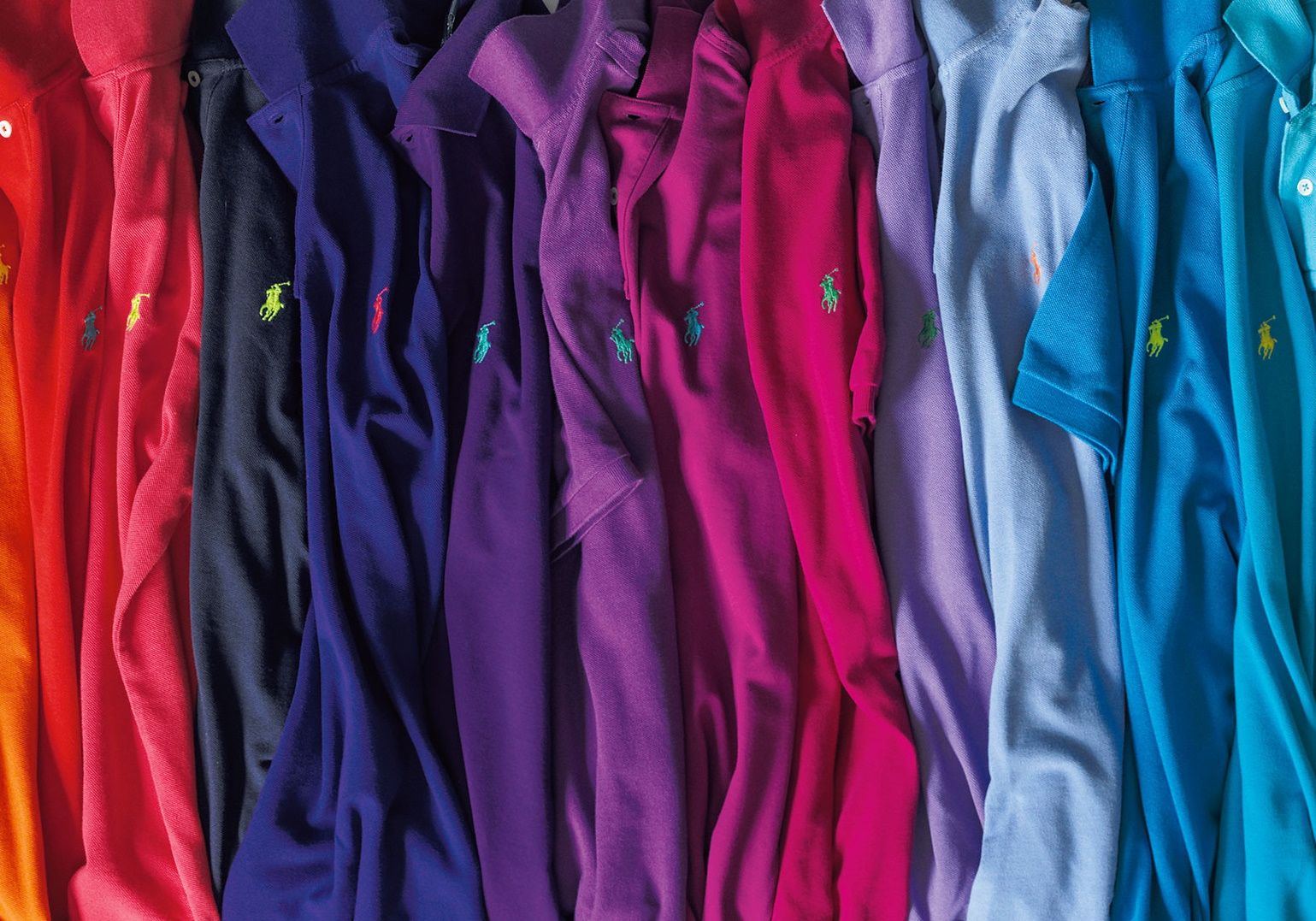The image features a side view of an array of Ralph Lauren polo shirts meticulously arranged by color, creating a stunning gradient effect. From left to right, the spectrum starts with orange and moves through red, pink, dark navy, royal blue, dark purple, lighter purple, magenta, hot pink, lilac, periwinkle, sky blue, and teal. Each short-sleeved shirt sports a distinct logo on the upper left chest, depicting a man riding a horse and holding what appears to be a polo mallet, indicative of the brand's signature style. The collars line the top of the image, while the occasional sleeve peeks out, with the bottoms of the shirts barely visible due to their close, slightly scrunched arrangement. These shirts are neatly laid next to one another, providing a vibrant, cohesive display of various shades.